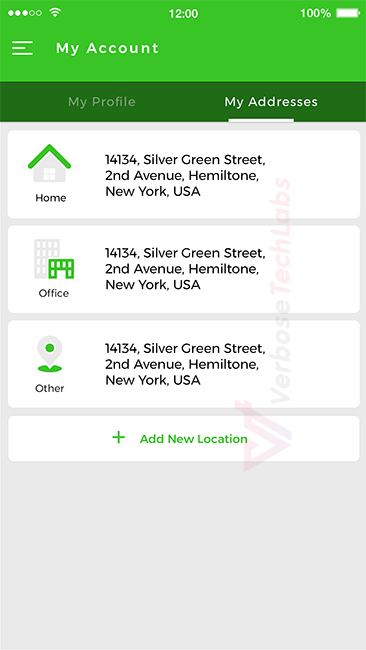Sure! Here is a highly detailed and cleaned-up descriptive caption for the given image:

---

The image appears to be a screenshot of a smartphone screen. At the very top, a light green section spans horizontally from left to right. Displayed in white font within this section, the time reads "12 o'clock" in the center, and on the right, the battery life indicator shows "100%".

Directly below this, on the left, there are three very thin horizontal lines. The top and bottom lines are of equal length, while the middle line is shorter. Positioned alongside these lines in white font, it states "My Account".

Beneath this, there is another thin banner, darker green in color. On the left side of this banner, in a grayed-out white font, it reads "My Profile". Next to it, on the right, it displays "My Addresses" in a brighter white font, and an underline emphasizes its selection.

Following this, the screen is divided into three interactive sections. On the leftmost section, an icon resembling the front of a single-family home, with a green roof, is displayed. Below the icon, the label "Home" is written in black font. To the right of this, a detailed address is listed in black font: "14134, Silver Green Street, 2nd Avenue, Hamilton, New York, USA."

The middle section shows an icon of a tall skyscraper office building, with a gray building in the background and a green one in front. Underneath this icon, the label "Office" is written, followed by the same address as above: "14134, Silver Green Street, 2nd Avenue, Hamilton, New York, USA."

The rightmost section has an icon that looks like a location pin, featuring a green dot in the center of a larger green circle. Below this icon, it reads "Other", accompanied by the same address once more: "14134, Silver Green Street, 2nd Avenue, Hamilton, New York, USA."

At the very bottom of the screen, a smaller section contains a green cross icon, next to the label "Add New Location". 

---